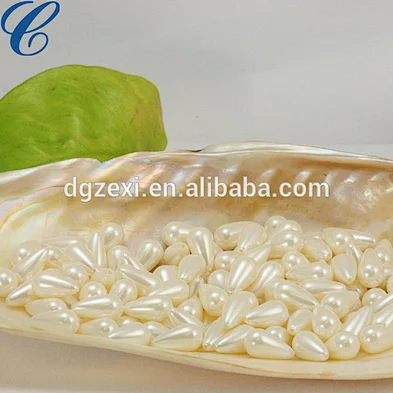This image features an advertisement for Alibaba, specifically showcasing a collection of artificial pearls. At the center of the image is a large, cream-colored shell filled with approximately 35 to 40 teardrop-shaped pearls, which are primarily purple but may also include greenish and white hues. These pearls are not arranged in a necklace but are scattered loosely within the shell. Behind the shell, there is a green leaf that seems to be part of a backdrop or banner. In the top left corner of the image, there is a blue, calligraphy-style letter "C." The web address, "dgzexi.en.alibaba.com," is prominently displayed in smaller, white standard font at the center. The pearls rest on what appears to be a silk or another smooth surface, adding to the luxurious appearance of the advertisement.